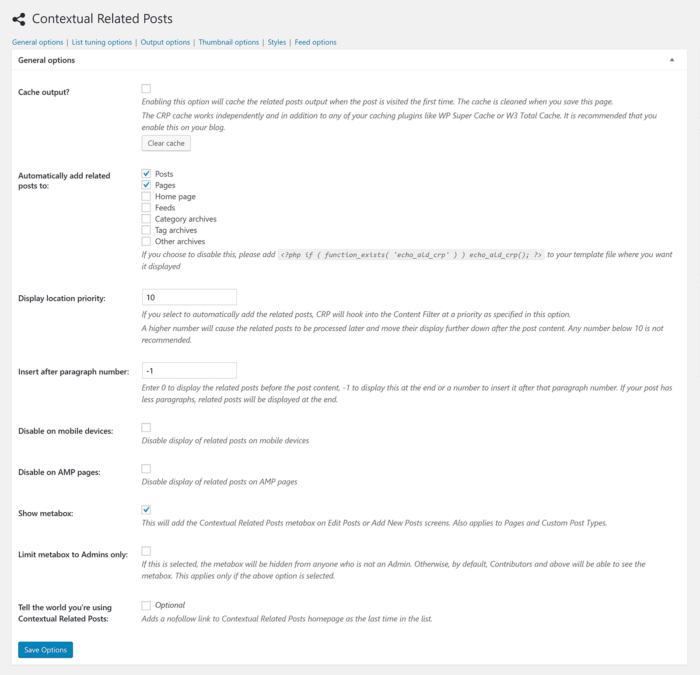The image displays a detailed view of a website's settings page, specifically for configuring related posts. The header, "Contextual Related Posts," appears against a light grey background, accompanied by a small logo to its left. Below the header, there are several small, blue subheadings such as "General Options," "List," "Turning Options," "Output Options," "Thumbnail Options," "Styles," and "Feed Options." The current focus is on the "General Options" page.

On the left side of the page, a vertical list of options is displayed in bold black text. These options include:

- General Options
- Cache Output
- Automatically Add Related Posts To
- Display Location Priority
- Insert After Paragraph Number
- Disable on Mobile Devices
- Disable on AMP Pages
- Show Metabox
- Limit Metabox to Admins Only
- Tell the World You’re Using Contextual Related Posts

At the very bottom of this list, there is a blue "Save Options" button.

To the right of each option title is a corresponding series of interactive elements, which can include single or multiple checkboxes, edit fields, some pre-filled with values, and others that can be enabled or disabled. These elements allow users to customize the functionality and appearance of related posts according to their preferences.